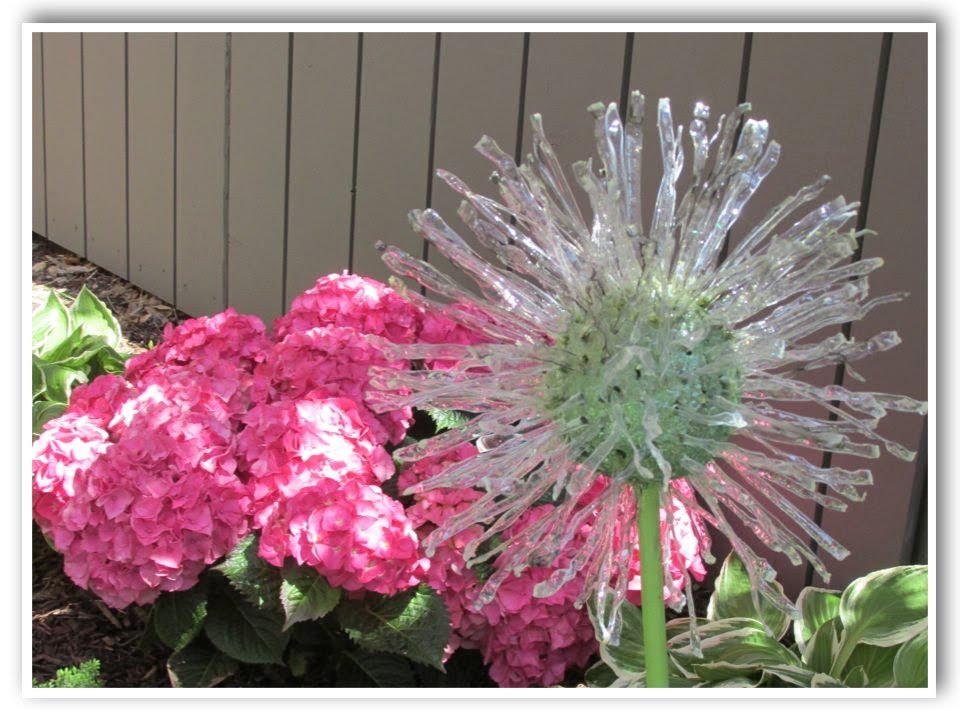This horizontally aligned rectangular image, bordered in white, captures a vibrant portion of an outdoor garden. Dominating the scene are brilliant pink flowers, likely hydrangeas or possibly carnations, adorned with lush green leaves. These flowers are clustered on the left side of the photo, adding a splash of tropical color to the setting. In contrast, a distinctive plant on the right features a light green stem topped with a spherical green center. From this center, translucent, narrow petals radiate in all directions, giving the flower a star-like appearance, almost as if its plastic-like components are crystallized. The garden's backdrop includes a gray wooden picket fence, visible only at the bottom due to the zoomed-in focus on the flora. Mulch covers the ground, adding a textural element to the garden scene, and some leaves with variegated white edges provide additional detail in the lower right corner. Overall, this image beautifully showcases the interplay of natural and possibly artificial elements in a serene garden setting.